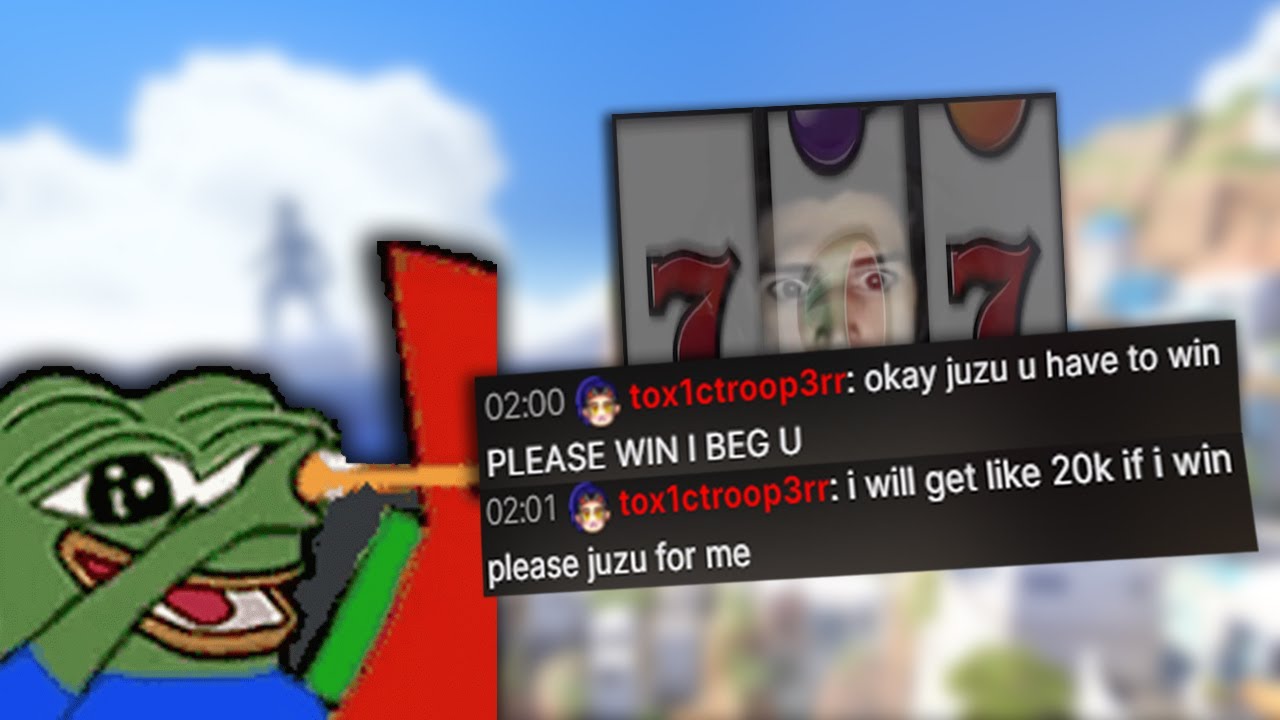In this unique and visually striking image, the primary focus is a close-up of a frog peering through a magnifying glass. The image seems to be displayed on a webpage. At the top of the image, text in various fonts and colors captures the viewer’s attention; it reads: "Two o'clock," followed by smaller text, "Tax 1 CT or See Troop 3 RR Okay Jiu-jitsu," culminating in bold white print, "Please win I beg you." 

Below, another timestamp "2:01" appears next to the same user's name in red, "Tax 1 See Troop 3 RR," with an impassioned plea stating, "I will get like 20k if I win Please juju for me." The background of the image is a blur of vibrant colors and shapes, evoking a sense of a bustling casino environment. Distinctly visible are slot machine reels featuring the number seven and various fruit symbols lined up as if in a game of chance.

Amidst this blend of digital and surreal elements, a faint human face watches intently, partially obscured by the vivid slot machine imagery. Behind it, a dreamlike, hazy blue sky and white clouds add a surreal atmosphere. The silhouette of a person standing in the clouds adds to the mystique, creating a contrast between the clarity of the foreground and the ethereal, almost abstract background.